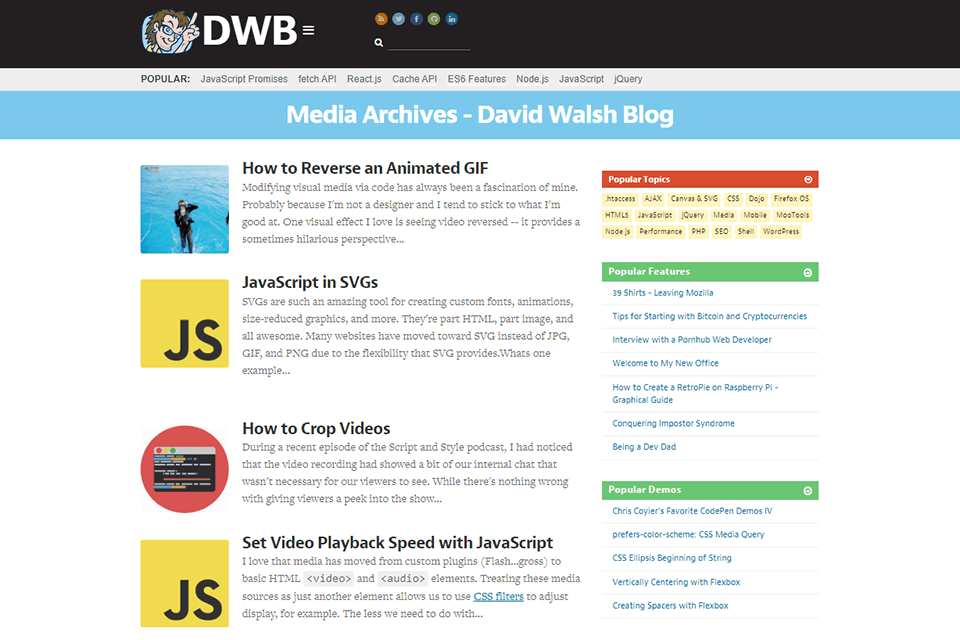**Caption:**

A screenshot of the David Walsh Blog (DWB) webpage. Prominently featured at the top left is the DWB logo next to a cartoonish illustration of a man with long brown hair, wearing glasses, an earring in his right ear, smiling contentedly, and holding up his pointer finger. Below this header, there is a black background section with icons for sharing the blog, and a search bar underneath. 

Directly beneath, it reads "Media Archives" followed by "David Walsh Blog", with four clickable article links:

1. **"How to Reverse an Animated GIF"**: This article explores the fascination of modifying visual media via code. Accompanying it is an image of a person in black attire, possibly in a swimming pool.
   
2. **"JavaScript and SVGs"**: Highlighted by a yellow box with black "JS" text.
   
3. **"How to Crop Videos"**: Features an image resembling a screenshot with a red background.
   
4. **"Set Video Playback Speed with JavaScript"**: Marked by the "JS" logo with a yellow background and some text difficult to read.

To the right of these articles are sections labeled "Popular Topics," "Popular Features," and "Popular Demos":

- **Popular Topics** include: Ajax, Canvas and SVG, CSS, Dojo, Firefox OS, HTML, JavaScript, jQuery, Media, Mobile, MooTools, Node.js, Performance, PHP, SEO, Shell, and WordPress.

- **Popular Features** showcase articles such as: 
   - "39 Shirts Leaving Mozilla"
   - "Tips for Starting with Bitcoin and Cryptocurrencies"
   - "Interview with the Pornhub Web Developer"
   - "Welcome to My New Office"
   - "How to Create a RetroPie on a Raspberry Pi: Graphical Guide"
   - "Conquering Imposter Syndrome"
   - "Being a Dev Dad"

- **Popular Demos** present items like:
   - Chris Coyier's favorite CodePen demos
   - "Prefers-Color-Scheme CSS Media Query"
   - "CSS Ellipsis Beginning of String"
   - "Vertically Centering with Flexbox"
   - "Creating Spacers with Flexbox".